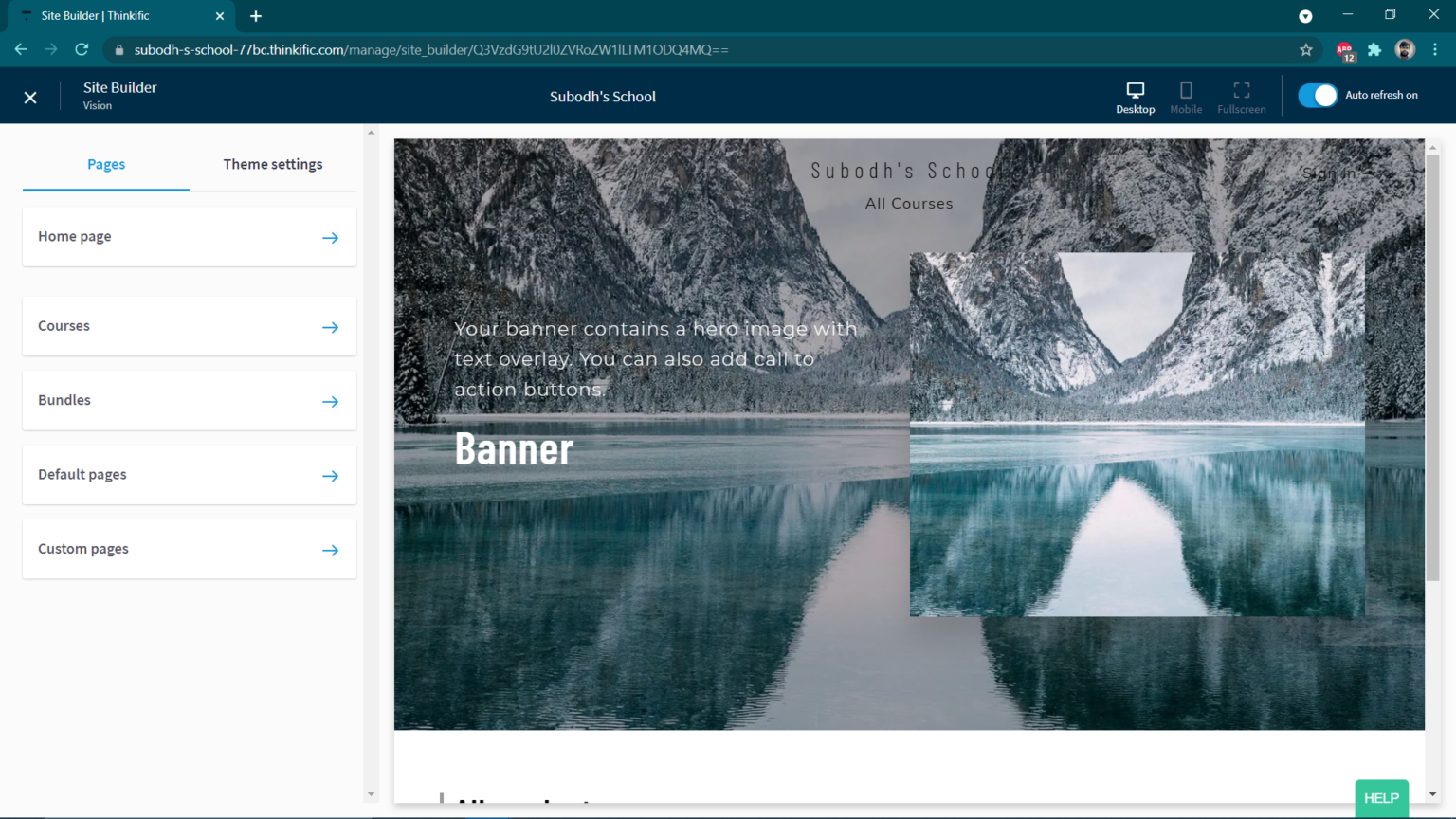**Descriptive Caption:**

A screenshot of a web design interface from the site builder Thrillik is displayed. The browser being used has a green theme, evident from the green tab and search bar at the top. Though the web address in the address bar is partially obscured and difficult to read, it is clear that the user is navigating within the Thrillik platform. On the left side of the tab, there is a distinctive 'X' icon for closing it.

Below this, the interface prominently shows the site builder with a project named "Subode School" indicated to the right of the builder's name. Various icons for previewing the website in different formats—desktop, mobile, and full-screen—are positioned near this. These icons are essential for testing the website's responsiveness across different device interfaces.

On the left-hand side of the interface, a vertical menu is visible with the "pages" section selected, allowing the user to manage and navigate through different pages within the project. The overall interface is designed efficiently for web development, with tools neatly organized for ease of access.